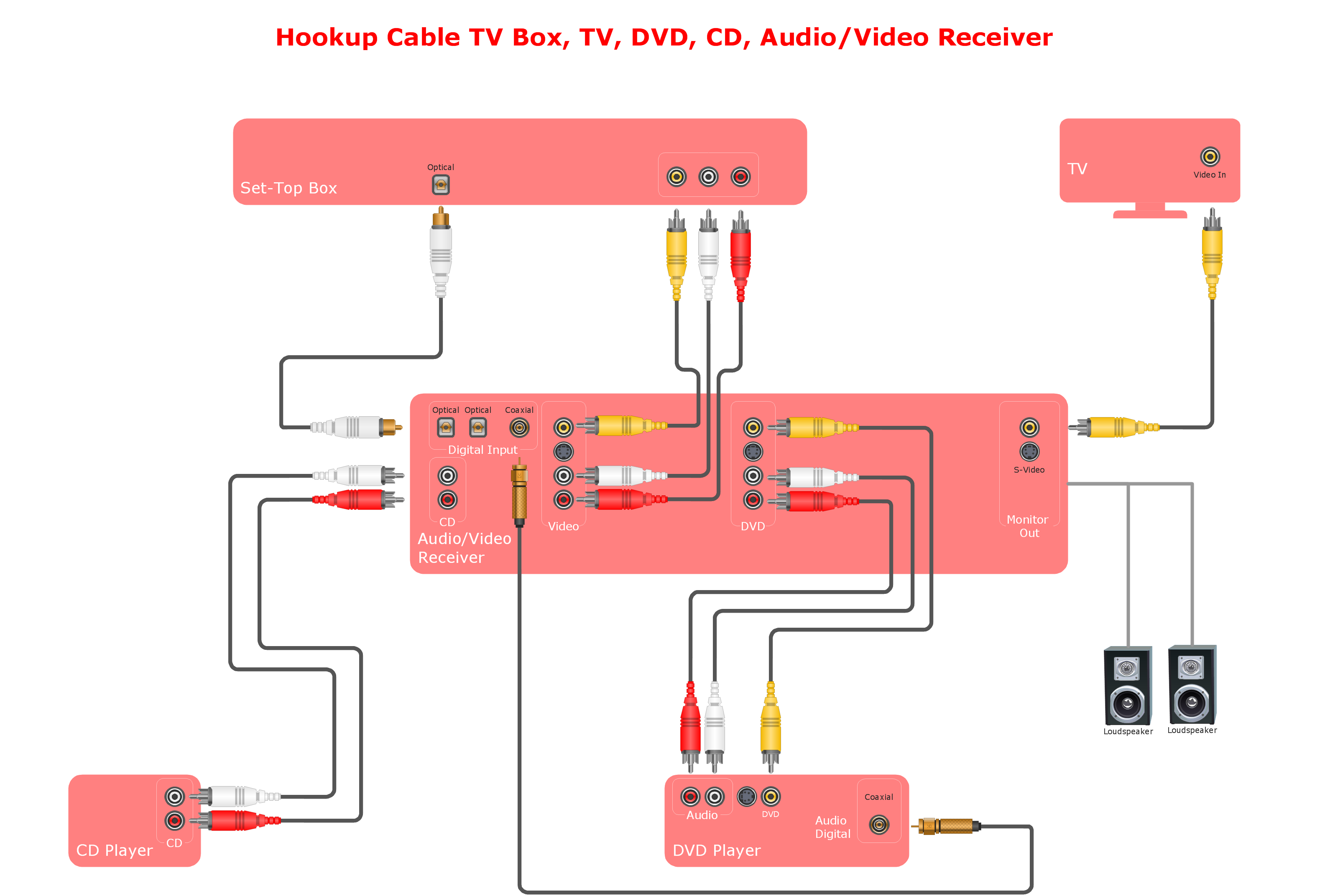This detailed product diagram is an informational guide from an instruction manual, showing how to properly hook up a cable TV box, TV, DVD player, CD player, and an audio-video receiver. The image consists of several pinkish-red rectangles, each representing a different device: a set-top box, the back of a TV, an audio-video receiver, a CD player, and a DVD player. Situated on the right side is also a diagram of two large speakers, which are wired up to the receiver. AV cables with yellow, white, and red plugs clearly indicate where each connection should be made on the devices. This cohesive blueprint provides a clear visual guide for setting up your entire audio-visual entertainment system, ensuring all components are correctly connected and operational.